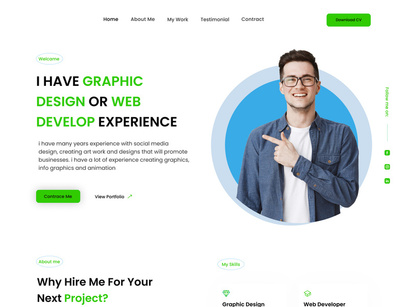On a clean white background, centered near the top in black text, are the menu options: "Home," "About Me," "My Work," "Testimonial," and "Contact." On the right-hand side, within a green rectangle, black text reads "Download CV."

Beneath this, still on a white background, there is a gray circle situated to the left with the green word "Welcome" inside it. Adjacent to this, in black text, it says "I Have," followed by green text listing skills: "Graphic Design," "Web Design," and "Experiences." Below these headings, a paragraph in black text reads: "I have many years of experience with social media design, creating artwork and designs that will promote businesses. I have extensive experience creating graphs, infographics, and animations."

On the right-hand side, there is an illustration of a man within a gray, blue, and white circle. He is pointing to the left. The man is depicted as a white individual wearing black glasses, a blue jean jacket over a white shirt, and has black hair and a blue shirt.

At the bottom left-hand side, there is a section titled "Why Hire Me for Your Next Project," offering reasons to consider the individual for prospective projects.